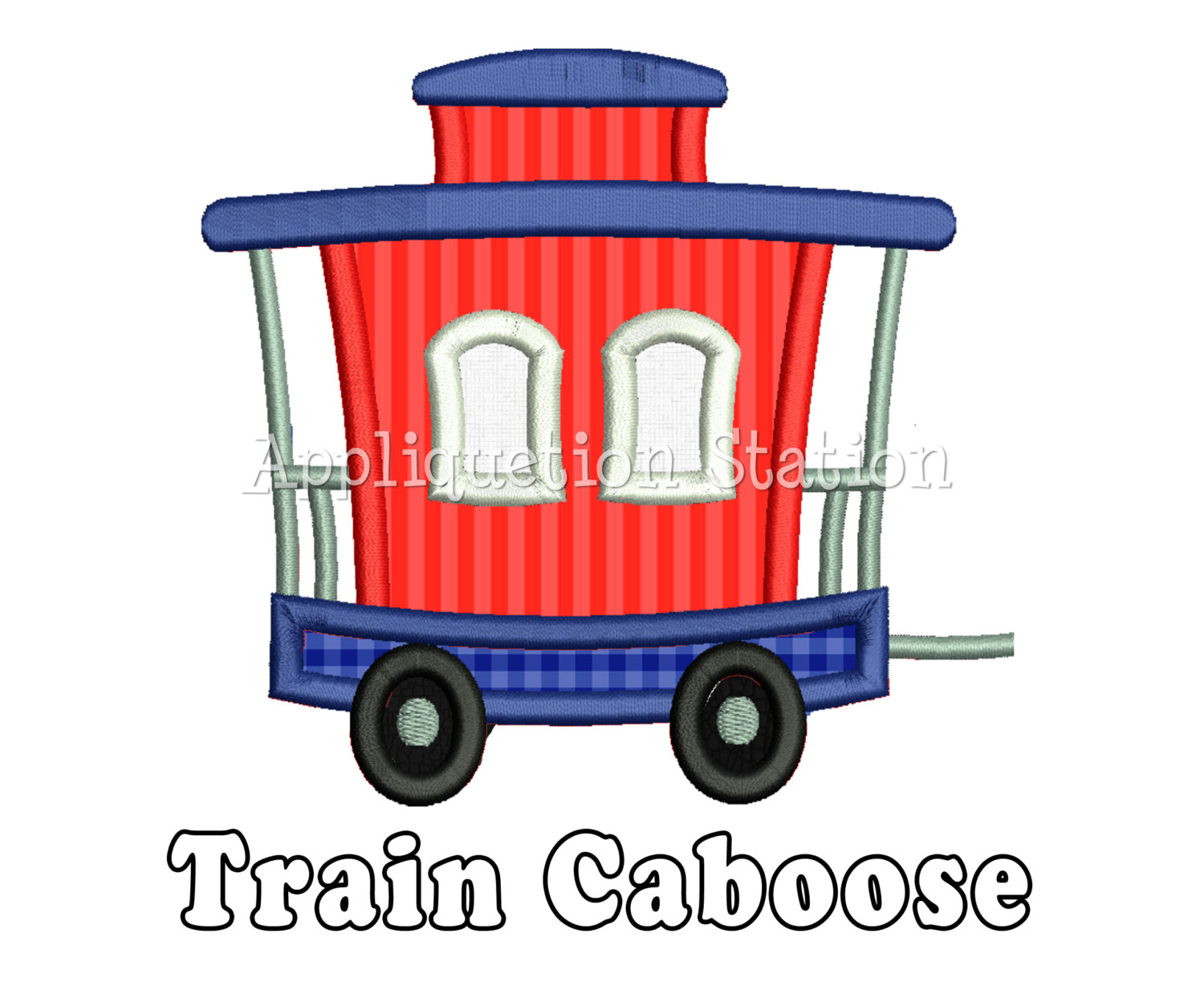This detailed illustration features a cartoon-style train caboose characterized by its vertical red and pink-red stripes. The caboose's primitive and blocky graphic elements are softened with a light fabric texture. Prominent blue accents appear at the top and bottom of the caboose, with the top portion layered in alternating blue and red sections. The two windows are pillowy in appearance, white with fabric-like texture and bordered edges. The wheels, depicted in concentric circles of charcoal gray, black, and silver, also exhibit a fabric texture. Silver poles extend vertically along the caboose, connecting it to an unseen part of the train. In the lower portion of the image, white text with a black border reads "train caboose." Additionally, the graphic features a watermark that says "Application Station" across the center. The background is purely white, emphasizing the vibrant colors and playful design of the caboose.